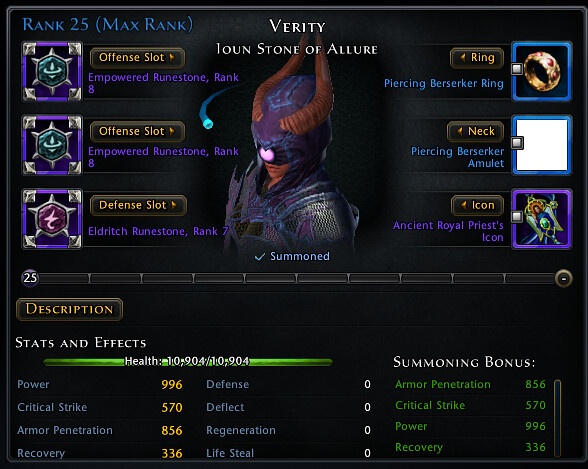The image is a detailed screen capture of a video game character stats page. Set against a black background, the top section prominently displays "Verity" and "I own Stone of Allure," with "Rank 25 Max Rank" on the upper left. The central figure is a character clad in gray armor with blue accents, sporting a helmet with two brown horns. The character's face is partially illuminated, showing lips beneath a light. 

On the left side, vertical text specifies "Offense Slot Empowered Runestone Rank 8" and "Defense Slot Eldritch Runestone Rank 7." Adjacent to them are controls labeled "Orange Slot," "Offense Slot," and "Defense Slot," highlighted in orange text. Below these controls lies an orange button marked "Description," followed by "Stats and Effects."

The right side lists "Ring Piercer Berserker Ring," "Neck Piercing Berserker Amulet," and "Icon Ancient Royal Priest's Icon," with a horizontal progress bar beneath. Further down, it shows detailed categories such as Power, Critical Strike, Armor Penetration, Recovery, Health, Defense, Deflect, Regeneration, Life Steal, and Summoning Bonus, with corresponding numerical statistics. 

Overall, the page meticulously outlines the character's equipment, attributes, and additional bonuses, indicating a high level of customization and character detail within the game.